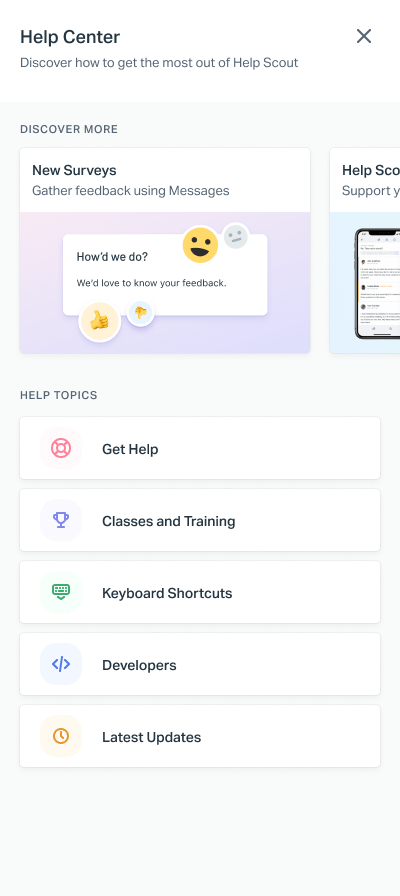This image is a screenshot of a website displayed on a smartphone, evidenced by its tall, narrow, vertically-oriented layout. The top of the screen features a pop-up menu labeled "Help Center" with a message prompting users to "Discover how to get the most out of Help Scout." This menu can be closed by tapping a small 'X' icon to reveal more of the page.

Directly below, the page invites users to explore various features with headings like "Discover More," "New Surveys," and "Gather Feedback Using Messages." An example under "Gather Feedback Using Messages" includes a prompt that says "How'd we do?" accompanied by emojis and thumbs-up icons, suggesting interactive feedback options. The layout allows for sideways scrolling to reveal additional yet partially obscured options, one of which hints at "Help SCO Support Y."

Beneath this section, several clickable options are presented in bar form. These include "Get Help," "Classes and Training," "Keyboard Shortcuts," "Developers," and "Latest Updates." Each bar likely directs users to specific help topics or resources. The screenshot appears to have been taken in a standard, non-dark mode setting, but it's unclear whether it's from an Android or iOS device as no distinct platform elements are visible.

Overall, the screenshot showcases the Help Center section of an application designed to assist users in utilizing its features and accessing support and resources.